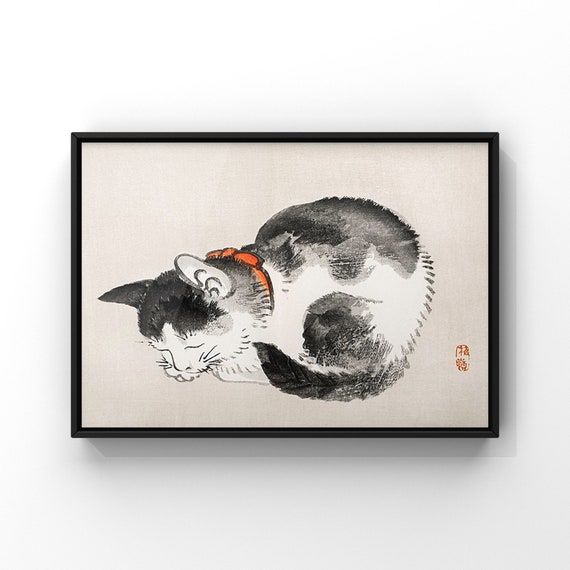This image features a framed piece of wall art, presented in a square format with a black border around it. The artwork, possibly a watercolor or marker drawing, depicts a black and white cat in a realistic, photographic style set against a light gray background. The cat, appearing almost lifelike, is crouched on all fours, its body predominantly white with black patches on the top of its head, back, upper legs, and the tip of its tail. The tail curls forward towards the neck, adding a dynamic feel to the composition. The cat’s head is angled downward, facing the bottom left corner of the artwork, while the body faces the left and the back faces the right side. It wears a distinctive red collar, buckled at the back of its neck. To the right of the image, there is a small signature in red, adding a subtle touch of color to the otherwise grayscale background.